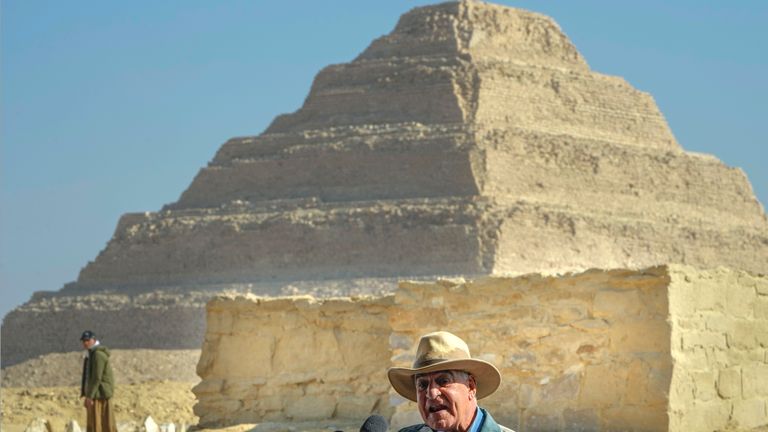The photograph, taken outdoors in Egypt, showcases a colossal and ancient, stepped pyramid rising majestically in the background. The pyramid, made from light brown or yellow stones, creates a dramatic and dusty atmosphere, likely from the surrounding sand. The sky above is clear and blue, adding to the arid, sunlit setting. In the immediate foreground stands an elderly man, possibly an archaeologist or researcher, with a weathered face and expressive eyes, mid-speech as he holds a press conference. He dons a dirty white or khaki cowboy-style hat that shades his face from the intense sun, and he wears a blue shirt. Just in front of him, the top of a black microphone is visible. To the left, another man, wearing a green jacket, brown pants, and a ball cap, stands further back, turned to the left, showing his left profile as he appears to listen attentively to the speaker.